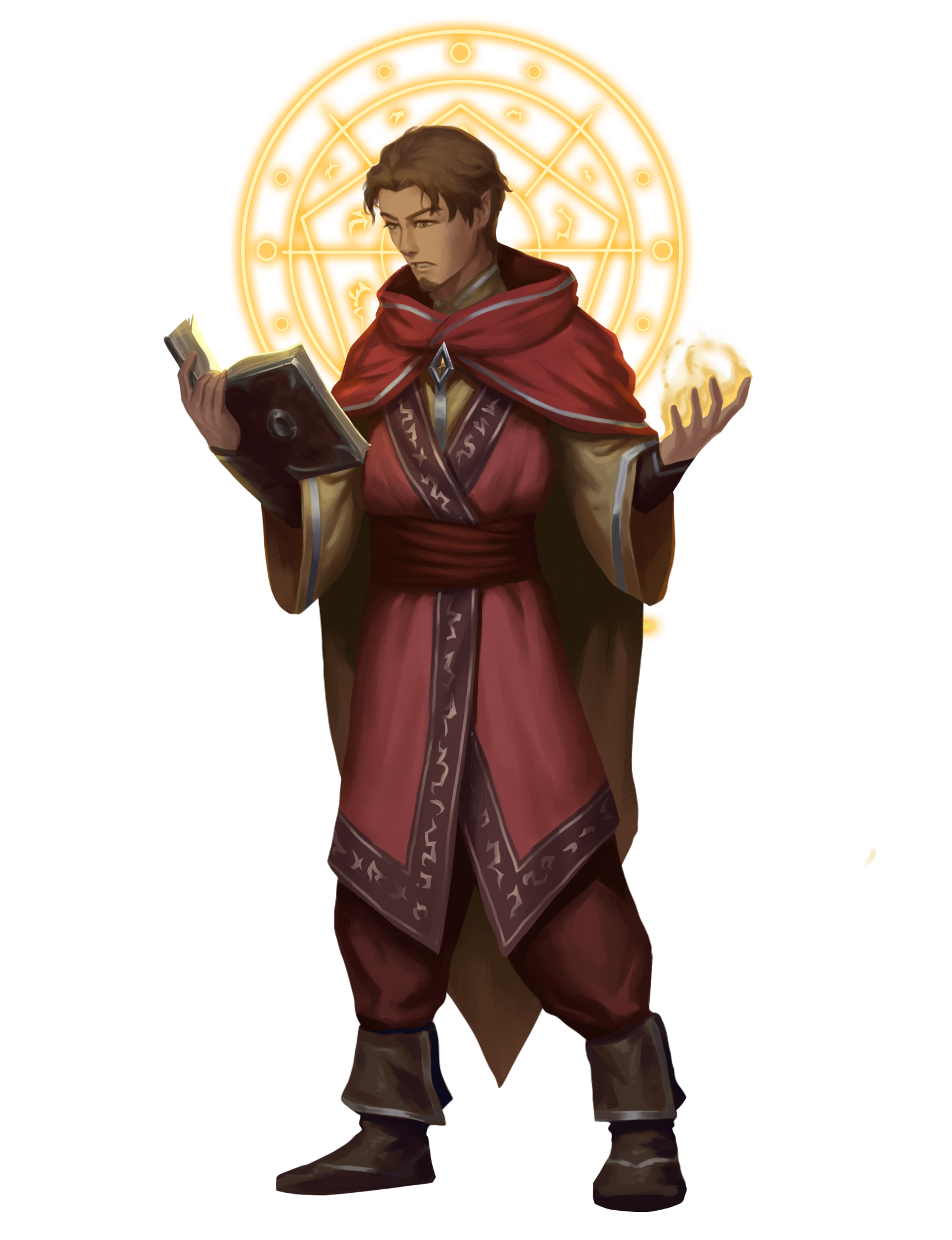This image is a highly detailed digital illustration, likely created with a stylus or pen tablet, depicting a male wizard or mage character. The figure appears to be around 30 years old, featuring short brown hair and a small goatee, with the rest of his face clean-shaven. He has pointed elf-like ears, adding a fantastical element to his appearance. 

The wizard is attired in medieval-style clothing, predominantly in shades of red and brown. He wears a striking red cape fastened at the collar, which drapes over a pinkish tunic sashed at the waist. His pants are balloon-like and similarly colored, complemented by brown boots that have rolled-down cuffs giving them a soft, worn appearance. Underneath the robe, there appears to be a yellowish-golden wizard shirt with wide sleeve openings, adorned with silver stripes at the ends, facilitating ease in casting spells.

The character is engrossed in a spell-casting process, as indicated by his focused gaze on a book held in his right hand, while a flame or fireball hovers above his left palm. This magical scene is further emphasized by a glowing golden circle, complete with intricate symbols, positioned behind him. The backdrop resembles a stained glass window without the glass, rendered in yellow and white hues, creating a mystical ambiance. Overall, this meticulously hand-drawn illustration serves as a compelling piece of character design or concept art, vividly capturing the essence of a spell-casting wizard.